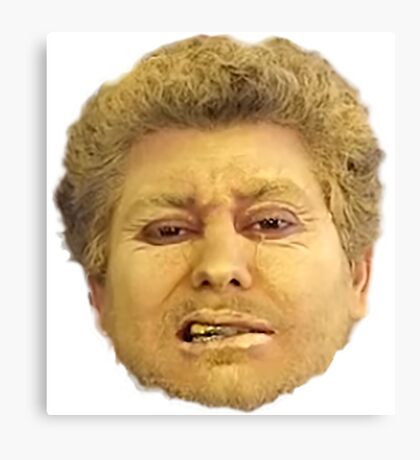The image depicts a head that appears to be digitally generated or heavily edited. It features a man whose face and hair are covered in a golden-brown, muddy texture, giving an overall impression of yellow paint. The complexion around his eyes remains untouched, suggesting he squinted tightly during the process, resulting in unpainted creases and darker circles around his eyes. His eyes are reddish-brown and his thick, curly brown hair is similarly coated in the same mud-like substance. The man is sporting a crooked grin, revealing a set of gold teeth, which adds to the odd and almost unsettling expression on his face. The background seamlessly transitions from a light grayish outer border to a white central area.